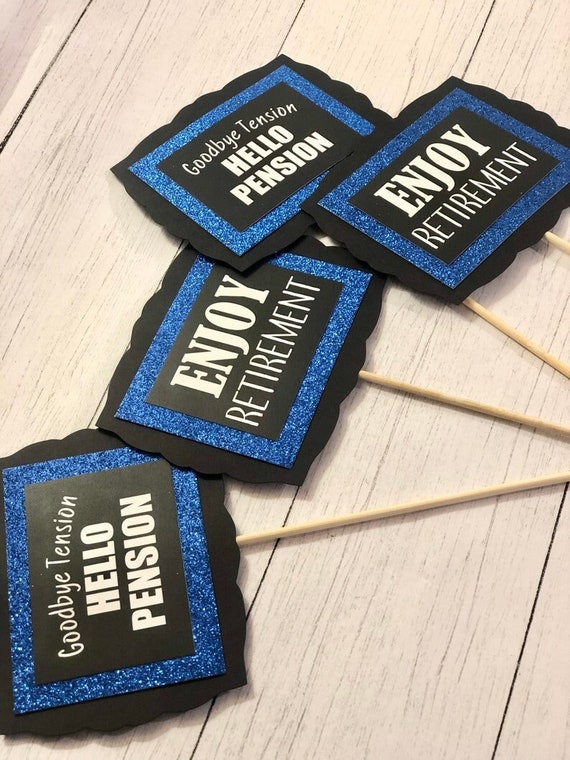The image displays a collection of four handmade signs, intricately crafted for a retirement celebration. Each sign is mounted on thin, round wooden sticks, arranged in a fan formation on a surface that appears to be made of bleached or light tan wood, with visible wood grain lines. The signs share a uniform design theme: a black wavy-edged border surrounding a sparkly blue background, overlaid with a black rectangle bearing bold white text. Two of the signs state "Goodbye Tension, Hello Pension," while the other two read "Enjoy Retirement."